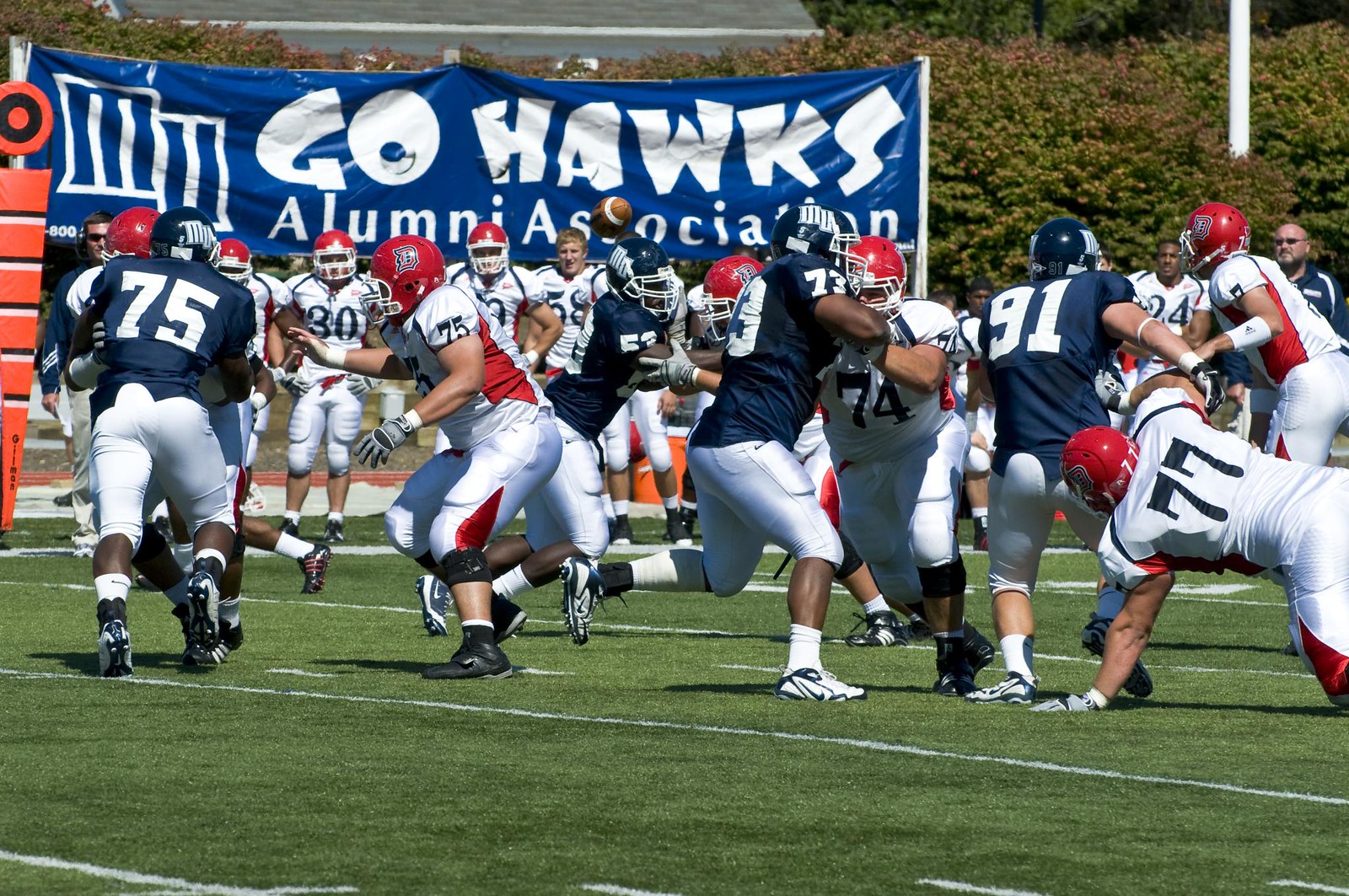This dynamic photograph captures the intensity of a football game between two teams, one in white and red jerseys with red helmets, and the other in white and blue uniforms with blue helmets. In the midst of a running play, the football is airborne as players from the offensive team attempt to evade tackles. The vibrant green field is marked with white lines and bordered by a tall line of bushes. On the left side, near the top, a distinctive orange marker with a bull's-eye symbol and blue and white lines is visible. Spectators, including players and a coach, line the sidelines, all under the watchful eyes of the referee holding the marker. A large blue banner that reads "Go Hawks Alumni Association" stretches across the background, adding to the spirited atmosphere. The scene, bathed in daylight, is dominated by hues of blue, white, green, and red, encapsulating the competitive energy of the game.